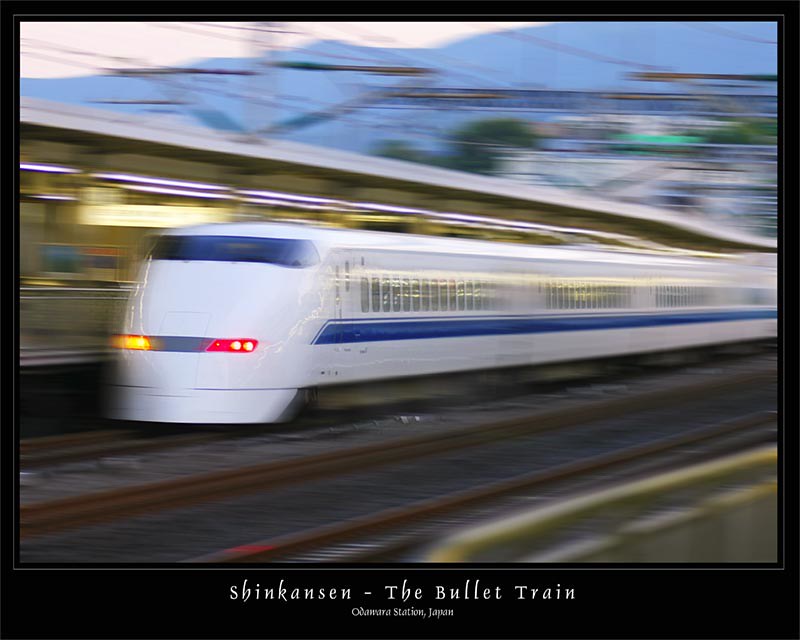The image is a poster styled in the popular 90s and early 2000s motivational format. It features a prominent black border with white text at the bottom center that reads "Shinkansen - The Bullet Train" and below it, in smaller font, "Odawara Station, Japan." The central portion of the image captures a white Shinkansen train, distinguished by a blue stripe running along its side and numerous windows. The train, traveling at high speed, appears heavily blurred, emphasizing its rapid movement as intended by the artist.

The backdrop includes a brownish mountain range in the upper part of the image, indicating a scenic but motion-filled environment. Towards the right, green trees and white buildings add depth to the scene. In the mid-ground, there is a station platform with a white roof and long fluorescent lights, illuminating the area. The foreground showcases two rust-colored tracks, along with a small grey concrete pillar at the bottom right corner. The sunlight and a somewhat clear blue sky suggest that the photo was taken during the day.